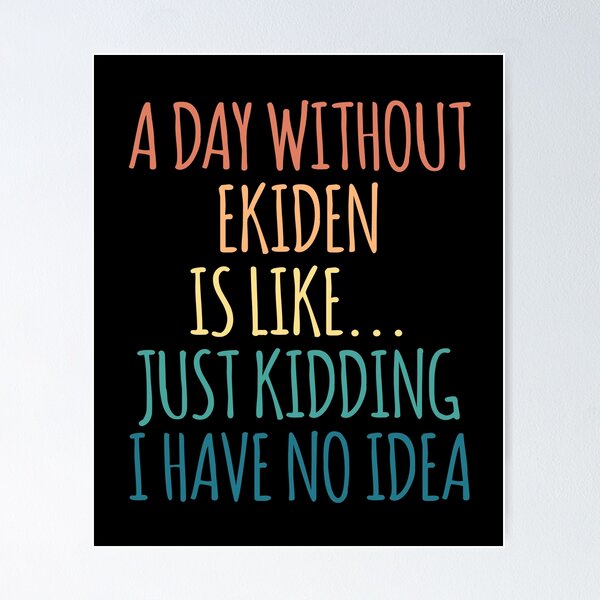The image features a vertical black rectangle set against a white or off-white background. Text in various colors is displayed on the black rectangle. At the top, the phrase "A day without Echidin is like..." is written, followed by "Just kidding. I have no idea." The word "Echidin" is spelled E-K-I-D-E-N. 

The text colors are as follows:
- "A day without" is in a light orange or reddish-orange color.
- "Echidin" is in shades of peach or orange.
- "Is like..." is written in a pale or light yellow.
- "Just kidding" appears in turquoise or aqua.
- "I have no idea" is written in a standard or sky blue color.

The font across the text is curvy or slightly slanted, giving the impression of a playful or humorous tone, suggesting it could be the cover of a book or a humorous print.